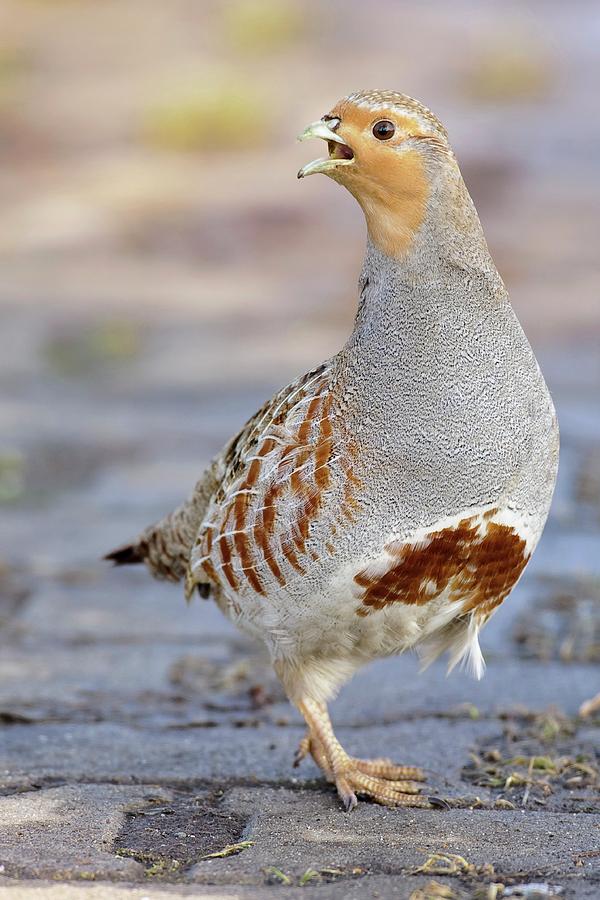The vertical rectangular image captures a detailed close-up of a small bird standing on a brick surface with scattered hay and a bit of grass. The bird features a mixture of colors and textures across its body. Its face has orange coloring around the mouth and eyes, black eyes, and a neutral beige beak, giving it a distinctive look. The bird's body is primarily covered in gray feathers with black dots on white feathers, creating an almost skin-like appearance in some areas. Its neck has gray feathers, while the underbody showcases a mix of white and dark brown feathers, and even hints of blue and soft white. The bird's wings are adorned with white and brown stripes accompanied by some white lines, and its tail is a dark brown color. Its yellowish feet with talons point to the right as it appears to be standing on a concrete surface mixed with some grass. The bird's head is centered in the image, with its beak open as if cawing, directed to the left. The overall image is taken during the daytime with no text associated, capturing the bird's full body, detailed plumage, and the muted colors of its surroundings.